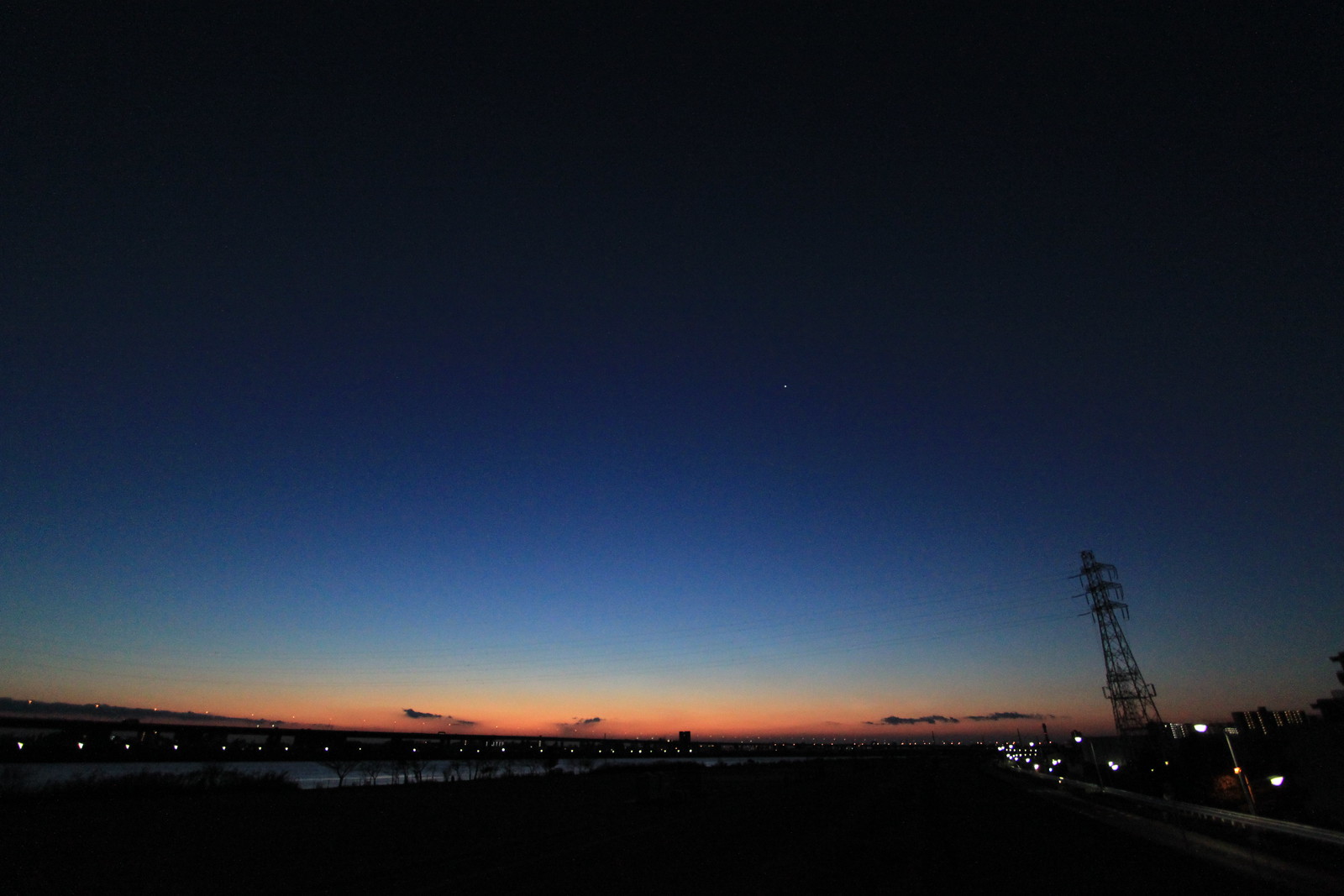The image portrays a cityscape at dusk with the sun recently set, painting the horizon in vivid hues of orange, pink, and red, while the upper part of the sky transitions into deep blue and black. A solitary, towering high-voltage power line stands prominently in the middle-right section, stretching its long wires into the distance. Adding to the scene’s tranquility, a lone star, likely Venus, twinkles brightly amidst the dark expanse above. Along the bottom of the image, faint lights suggest a structure, possibly a bridge or a canal barrier fence. A straight horizon line is dotted with small, thin clouds and distant lights, hinting at roads or cars that add a faint glimmer to the encompassing twilight.